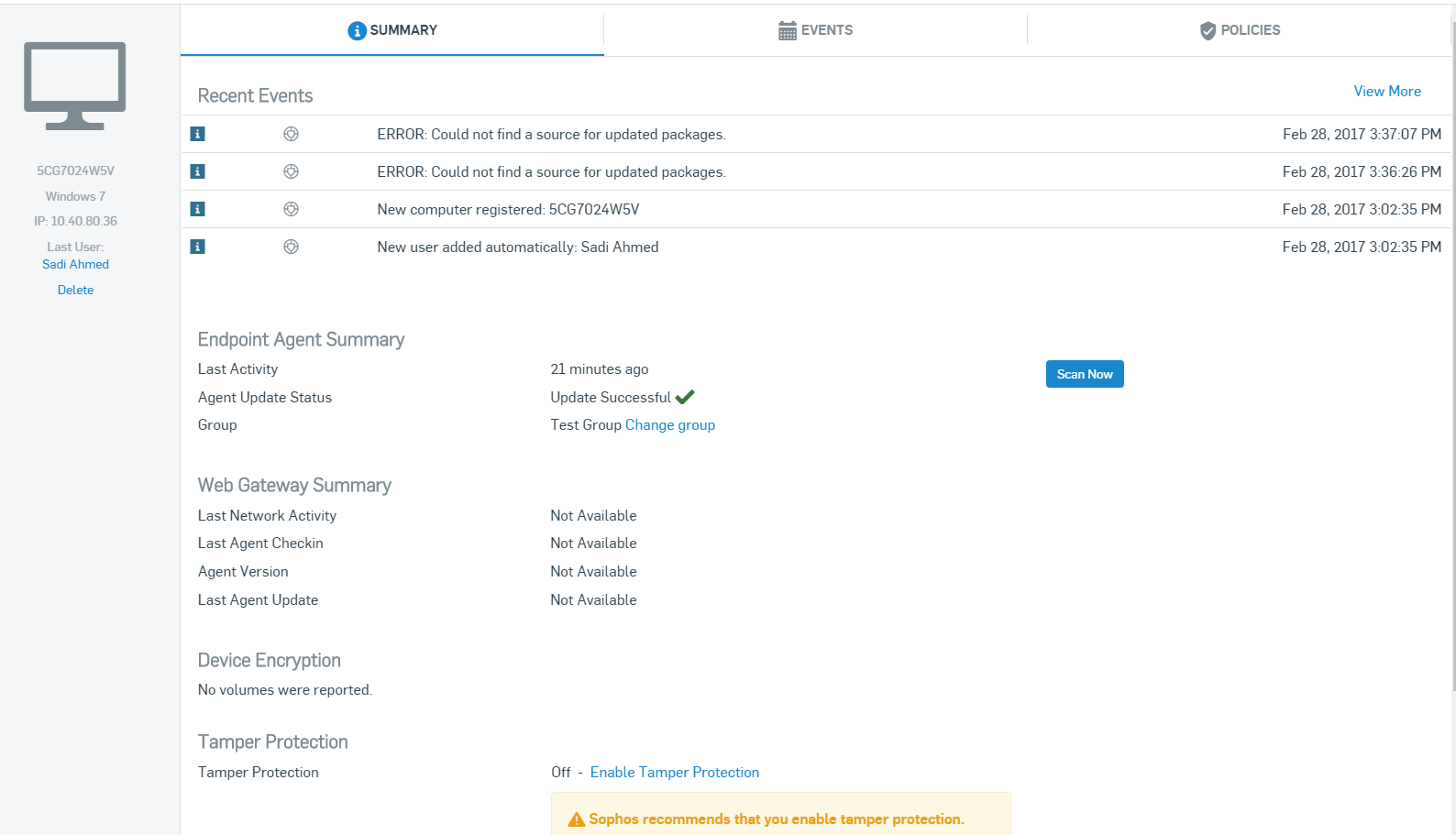This image is a detailed screenshot of an endpoint management application designed for the management and deployment of computers within a computer domain. The image provides a comprehensive overview of a specific Windows computer, displaying crucial technical details beneficial for IT support specialists.

On the left side of the page, a long vertical light gray box houses key information about the computer. At the top left corner of this box, the computer’s serial number or asset tag is clearly visible. Directly below this, in gray text, the operating system is identified as Windows 7. Additional details include the computer’s IP address and the last user who logged in, named Saadi Ahmed, which is highlighted in blue text. Beneath the user information, a blue "delete" link allows the option to remove the computer or its data from the system.

The central section of the page, set against a white background, presents extensive information about the computer. At the top of this section, three tabs labeled Summary, Events, and Policies are available, with the Summary tab highlighted in blue, indicating that it is the currently active view.

The Summary page provides an array of technical data essential for IT management. It includes recent events, an Endpoint Agent Summary, a Web Gateway Summary, details on device encryption, and tamper protection status. This information is critical for IT support, enabling them to monitor the computer’s network activity, manage its security features, and oversee its overall performance. Such data ensures that IT specialists can efficiently manage the computer, track its usage, and maintain its security within the network.